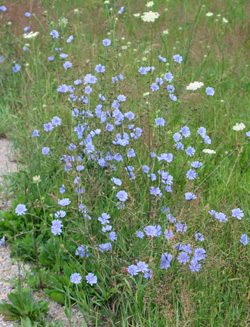This image is a color photograph capturing a field of wildflowers with both blue and white blossoms. Dominating the scene are numerous pale periwinkle blue flowers, believed to resemble forget-me-nots or cornflowers. These flowers, smaller with dark blue centers, populate tall green stems densely scattered throughout the frame. Interspersed among the blue flowers, taller white wildflowers, likely resembling daisies or Queen Anne's lace, punctuate the scene. The surrounding environment consists of mixed green and brown grasses and low-growing weeds. In the bottom left corner, pavement or concrete is partially visible, suggesting a border to this natural setting. Additionally, a dirt trail appears along the left edge, winding halfway down the photo and showcasing more green plants with protruding white blooms. The photo, slightly washed out and of moderate resolution, suggests an informal snapshot capturing a rich tapestry of wildflowers in a flourishing, untamed habitat.